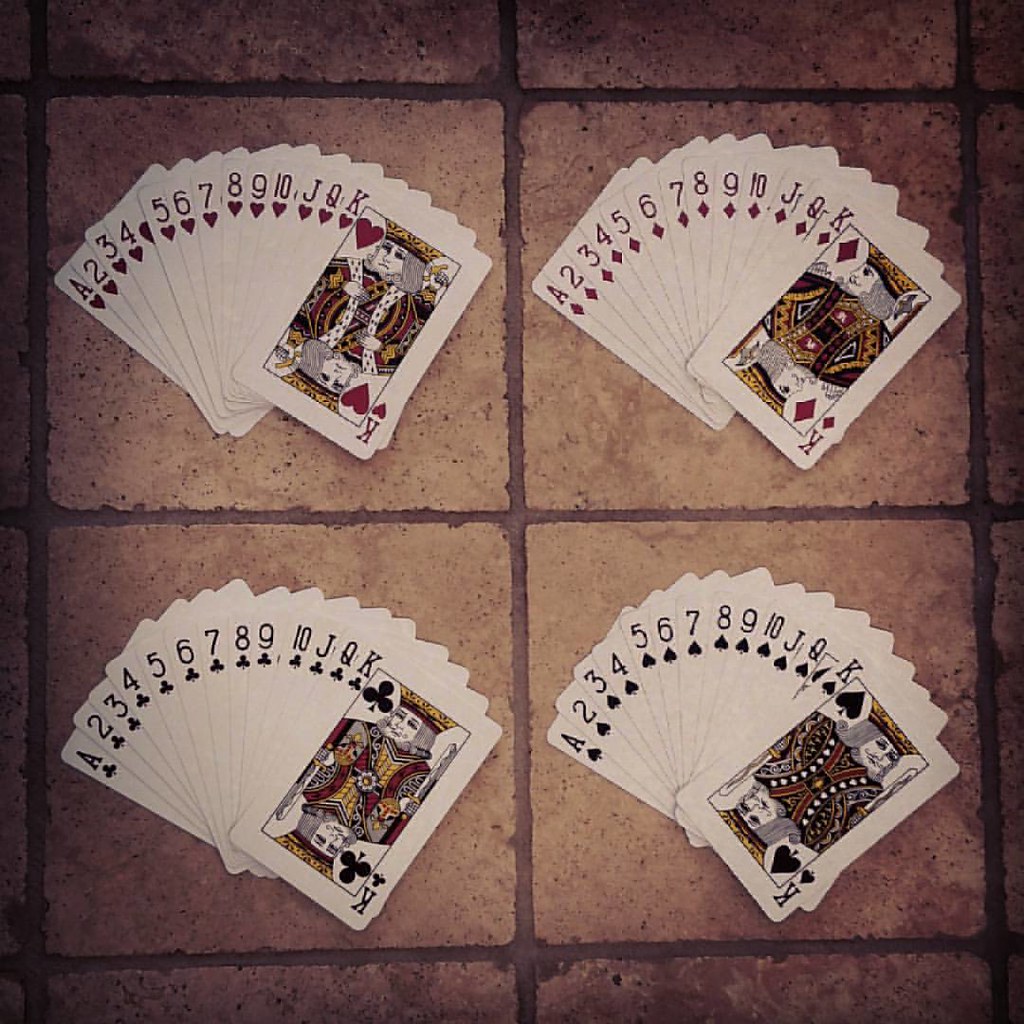This photograph showcases a section of a ceramic tile floor comprising four square tiles, each in a warm terracotta hue. The tiles are separated by dark brown grout lines, forming a distinct cross shape at the intersections. Spread out on each of the tiles are full suits of playing cards arranged in a fan pattern, mirroring how a person might hold them. The sequence of cards begins with the Ace on the left and progresses through to the King on the far right, with each suit meticulously ordered as follows: Hearts occupy the upper left tile, Diamonds are positioned on the upper right tile, Clubs are set on the lower left tile, and Spades are displayed on the lower right tile. The arrangement creates a visually pleasing, symmetrical layout. The playing cards are standard and unembellished, reinforcing the focus on the geometric and orderly aesthetic of the composition.